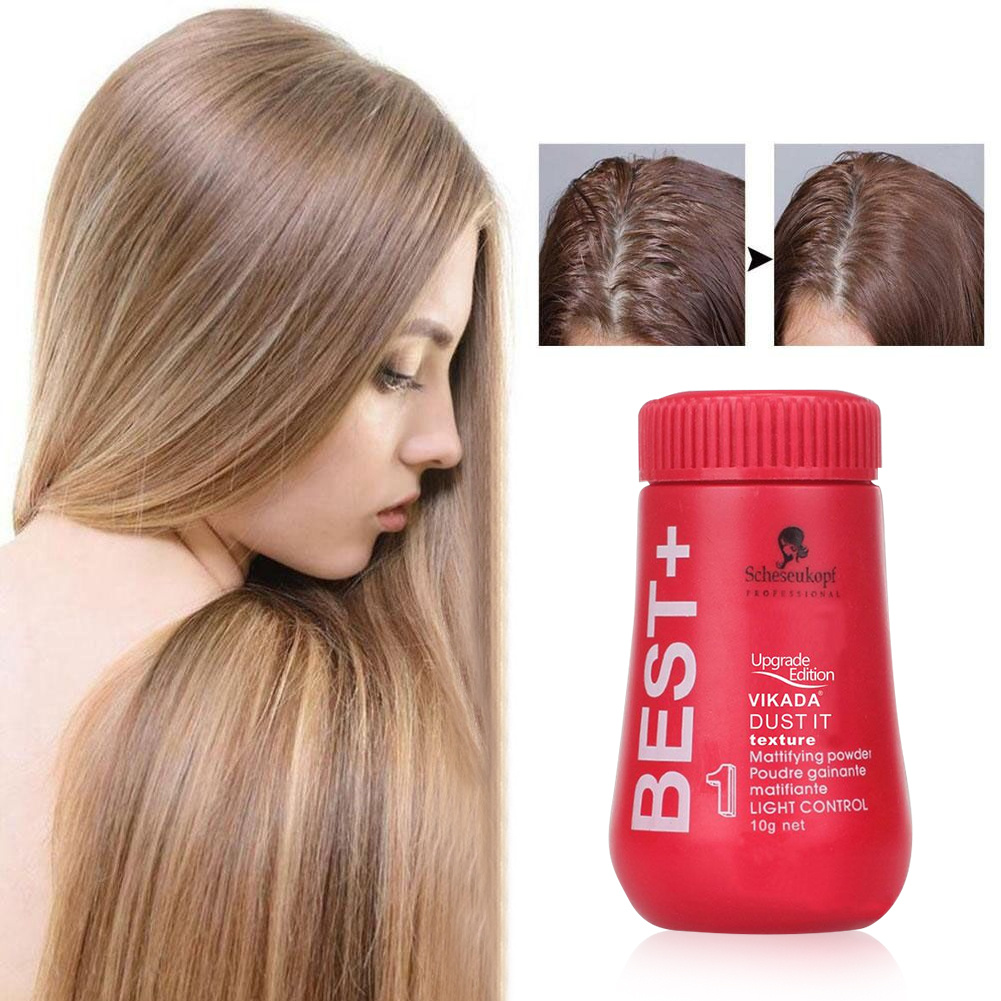This advertisement showcases the Best Plus Vicada Dust-It Mattifying Powder, a hair care product designed for light control and enhancing hair texture. The centerpiece is a striking red bottle with a screw-on top, prominently displaying a Schusskopf logo—a black profile head facing right, thicker at the base. The text includes "Upgrade Addiction" and details about the mattifying properties, with additional French text and the weight indicated as 10 grams. To the left, a young woman with long, light brown hair highlighted with blonde stands out. Her profile shows her looking downward, showcasing her flowing, well-maintained locks. At the top of the image, two small square pictures depict a noticeable transformation: one scalp appears whiter and messy, while the other looks neater and more refined, illustrating the product's effectiveness in managing hair appearance.